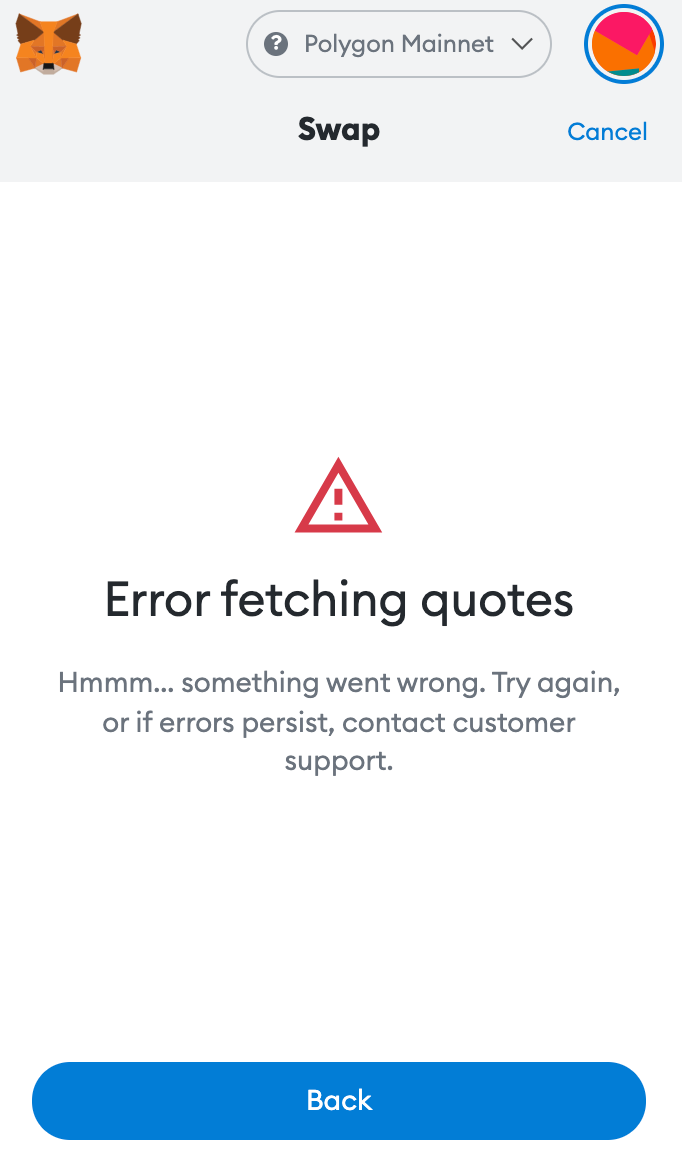Screenshot of an error message on a digital platform. In the top left corner, there's a fox-like icon. Next to it, a drop-down menu labeled 'Polygon Mainnet' is visible. Further to the right, a black button labeled 'Swap' and a blue 'Cancel' button are seen. Dominating the center of the image, a red warning sign is displayed with the message "Error fetching quotes." Following this, the text "Hmm, something went wrong. Try again or if error persists, contact customer support" is shown. At the very bottom, a long blue button with 'Back' written in white letters completes the screenshot.